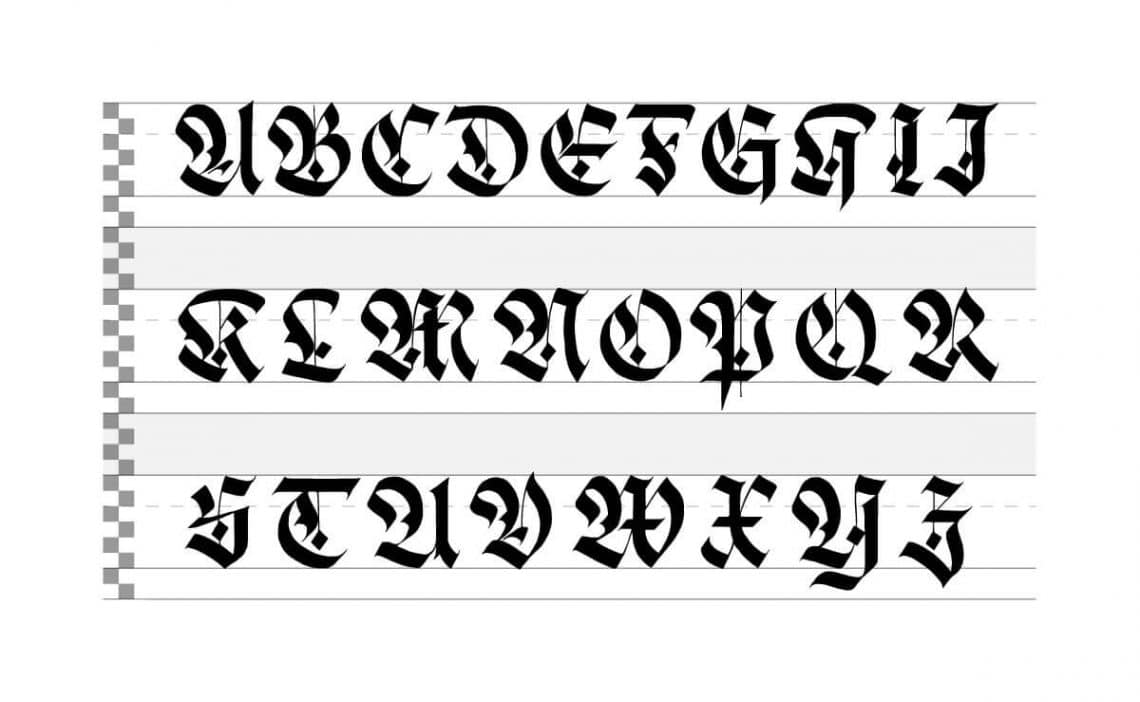The image is a computer graphic displaying the entire alphabet in a very ornate, medieval-style calligraphy font. The letters are arranged across three rows: the top row features A through J, the middle row runs from K to R, and the bottom row includes S through Z. The font is highly artistic and difficult to read, giving the letters an appearance reminiscent of ancient manuscripts. The text is in bold black, set against a background with light blue horizontal lines that resemble calligraphy practice guides. Along the left edge of the image, there's a vertical strip with a small white and gray checkerboard pattern, adding a distinctive decorative element.